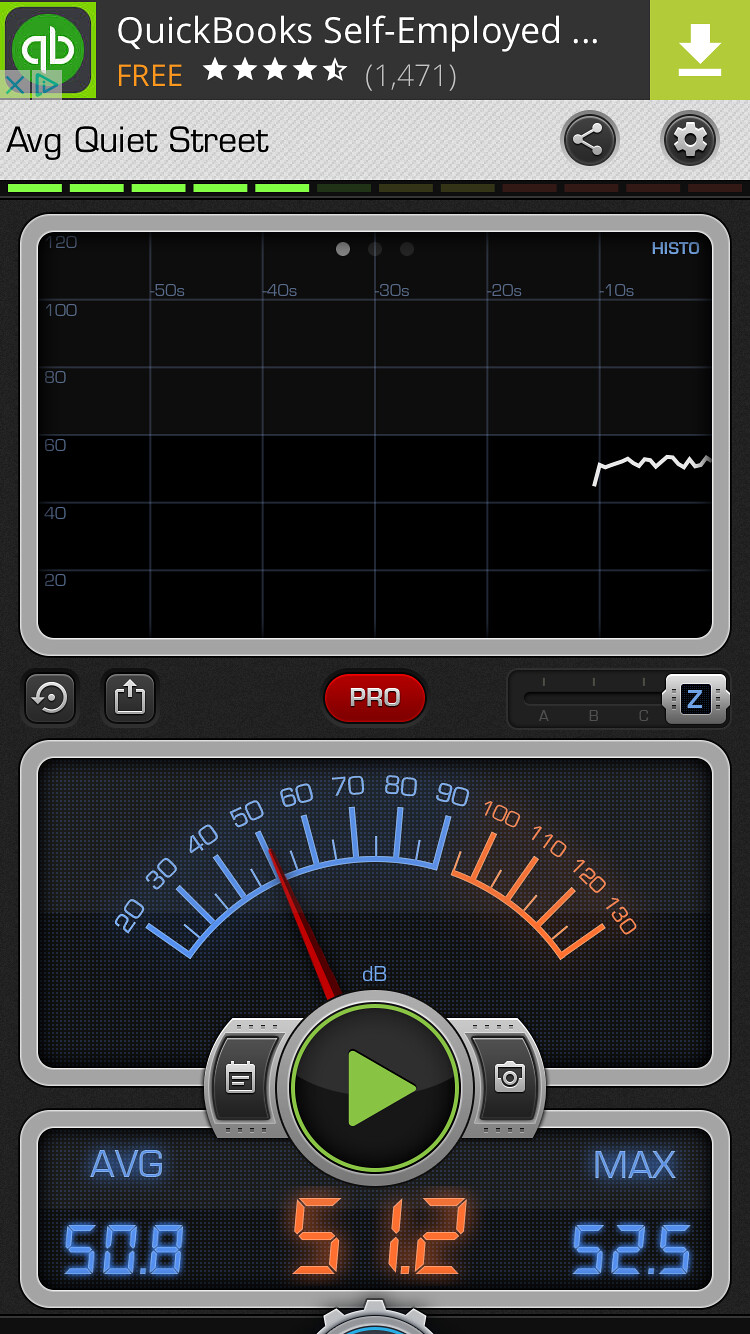This screenshot appears to be from a phone displaying an application with a primary gauge used to measure decibels, likely for noise levels. At the very top, there is a green banner ad for the QuickBooks Self-Employed app, rated at four and a half stars with 1,471 reviews. Below the ad, a gray banner with black text reads "Average Quiet Street," accompanied by share and settings icons in circles.

The main portion of the image is a dashboard on a black background. Centrally, there is a half-dial gauge indicating decibel levels, with the values ranging from 20 to 90 in blue and 100 to 130 in orange. This gauge is reminiscent of a speedometer, with a right-pointing green arrow in the center. Above the gauge, a red button labeled "Pro" can be seen. Above this is a black grid table, possibly displaying historical data.

At the bottom of the gauge, there are three digital displays with LED-style fonts showing numerical readouts: on the left, "50.8" in blue indicating the average; centered, "51.2" in larger red digits representing the current measurement; and on the right, "52.5" in blue denoting the maximum value recorded. Underneath these readouts, a large green play button suggests the functionality to start a new measurement.